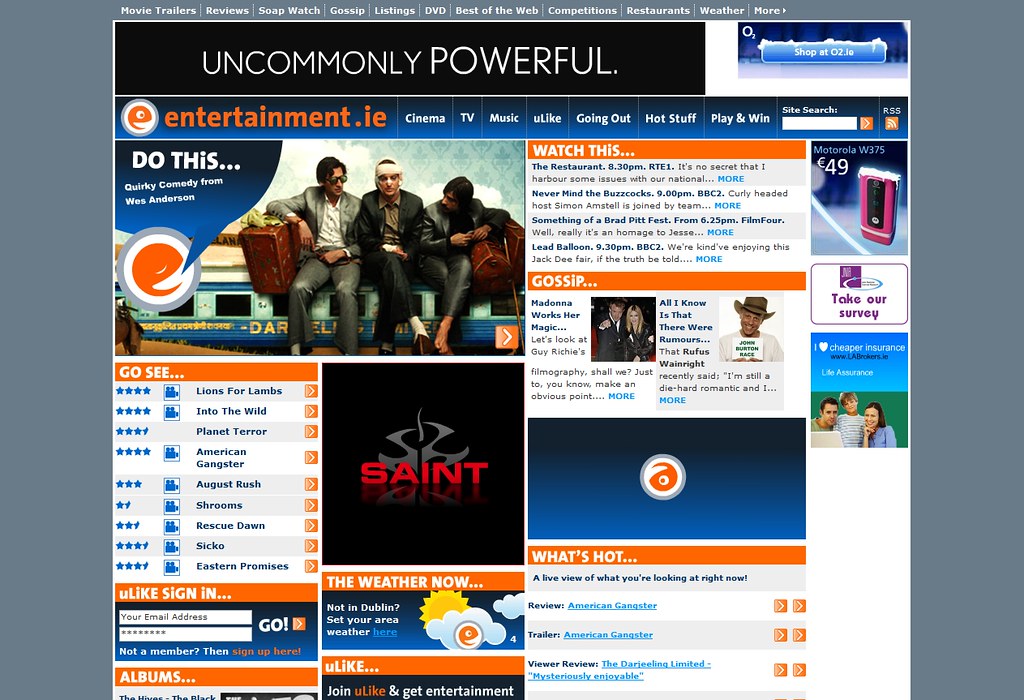The image showcases a detailed web page from Entertainment.ie, identifiable by its consistent orange theme and a recognizable logo of a stylized 'e' face enclosed in a circle. The dark gray outer border frames the page, which opens with a prominent navigation bar featuring options like Cinema, TV, Music, and Gossip, all in white font against a blue background. Aligned to the right of the navigation bar, there's a white search bar and an RSS feed icon.

Below the navigation bar, a striking black banner with white, all-caps text reads "UNCOMMONLY POWERFUL." Adjacent to this, on the upper right, a small rectangle promotes a shop at O2.io. Immediately beneath, there's an orange banner displaying the site’s name, Entertainment.ie.

The main body of the page is divided into several rectangular sections. To the left, beneath the Entertainment.ie banner, a section titled "Do This" includes a picture of three men sitting on a bench with luggage beside them, the middle man notably sporting a white head bandage. Just below, a "Go See" section lists various movie titles such as "Lions for Lambs," "American Gangster," and "Rescue Dawn," each accompanied by star ratings.

On the right-hand side, a section labeled "Watch This" precedes another titled "Gossip," which teems with text. Beneath these, a "What's Hot" section in an orange header lists trending items. Scattered advertisements, including a prominent one labeled "SAINT" in red against a black backdrop, accentuate the busy and information-rich layout of the page.